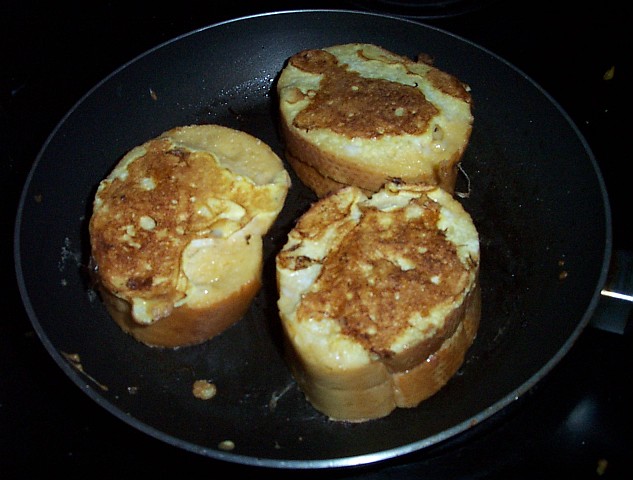This is a close-up photograph of a large, black, nonstick frying pan resting on what appears to be a glossy black glass cooktop. The pan contains five pieces of bread in total, forming three portions of what looks like French toast. Two of the portions consist of two pieces of smaller, French loaf bread stacked on top of each other, while the third portion is a single, thicker slice of bread. Each piece of bread appears to have been dipped in egg and fried, with the egg coating turning a dark, golden brown, almost overcooked, giving it a shiny, greasy appearance, likely due to the use of butter during cooking. The pan and its contents dominate most of the image, showcasing the rich, well-done texture of the toast and the distinct layering of the bread and egg mixture.